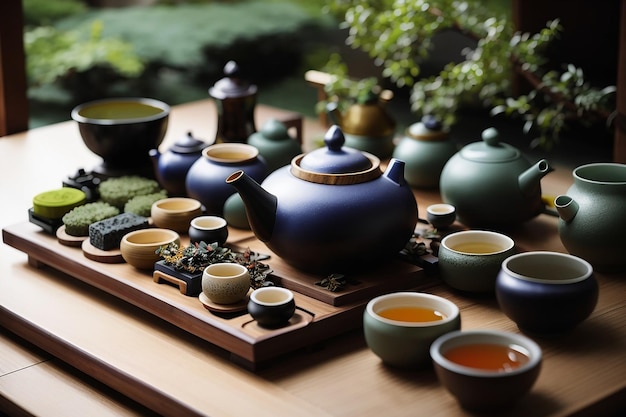The image depicts an intricate setup for a Japanese tea ceremony, arranged on a low, wooden table. Central to the composition is a large blue ceramic teapot, flanked by several wooden trays of varying sizes. The largest tray at the bottom holds the entire arrangement, while the upper trays present a meticulously organized display of teaware. On the top tray, there are four small bowls filled with different colored teas—gold, red, yellow, and another undetermined hue. Adjacent, there are two stout teapots, one green with a long narrow spout, and another darker-colored one. Smaller wooden trays within the arrangement contain tiny tasting bowls, some as small as shot glasses, suggestive of samples or different types of tea. Surrounding the teapots and bowls, the table is adorned with additional teapots and other pots, possibly for condiments like sugar. The setting is complemented by shiny green bushes in the backdrop, enhancing the serene atmosphere typical of a Japanese garden.